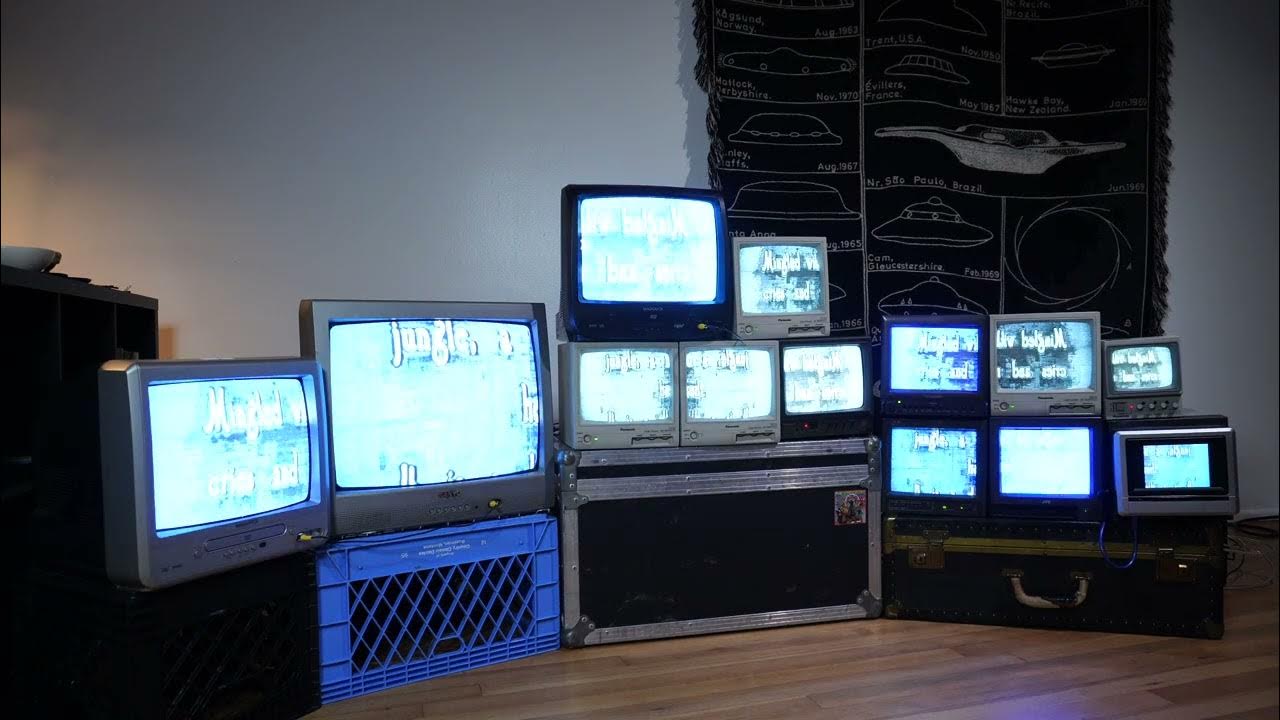The photograph is an indoor staged scene illuminated entirely by artificial light, capturing a room with a gray wall and a hardwood floor. Dominating the scene is an eclectic arrangement of 13 old television sets, all turned on, casting the primary light in the image. These TVs are precariously stacked on various objects, including metal boxes, suitcases, and plastic milk crates—one notably blue. The intricate formation includes three small TVs bearing larger and smaller TVs on top, and further groupings, such as five TVs stacked on a black trunk with a white handle and another set of six TVs atop another crate. The back wall features a black hanging banner or rug adorned with white diagrams of flying saucers, adding an eccentric touch to the otherwise chaotic display of vintage technology. This meticulously constructed tableau combines elements of nostalgia and otherworldliness, anchored by the contrasting wooden floor and the gray wall.